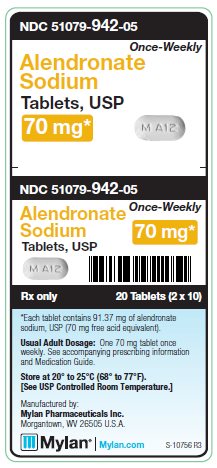The image shows a mobile-optimized webpage detailing a specific prescription medication. At the top, the label reads "NDC 51079-94205," indicating it's related to medication. The main section highlights "Alendronate Sodium Tablets, USP, 70 milligrams," prescribed for once-weekly administration. An image of the tablet, inscribed with "MA12," is displayed prominently.

Further details reveal the same information below, accompanied by another image of the "MA12" tablet and a barcode for scanning. A header states "RX only," signifying the medication requires a prescription, and specifies the package contains "20 tablets, 2x10."

Beneath this, the text notes that each tablet includes "91.37 milligrams of Alendronate Sodium, USP," and mentions the typical dosage is one 70 milligram tablet per week. Important directions are provided to consult additional prescribing information and the medication guide. The storage instruction advises keeping the medication at a temperature of 20 to 25 degrees Celsius.

The bottom section confirms the manufacturer as Mylan Pharmaceuticals, located in Morgantown, USA, and directs users to their website, mylan.com, for further details.